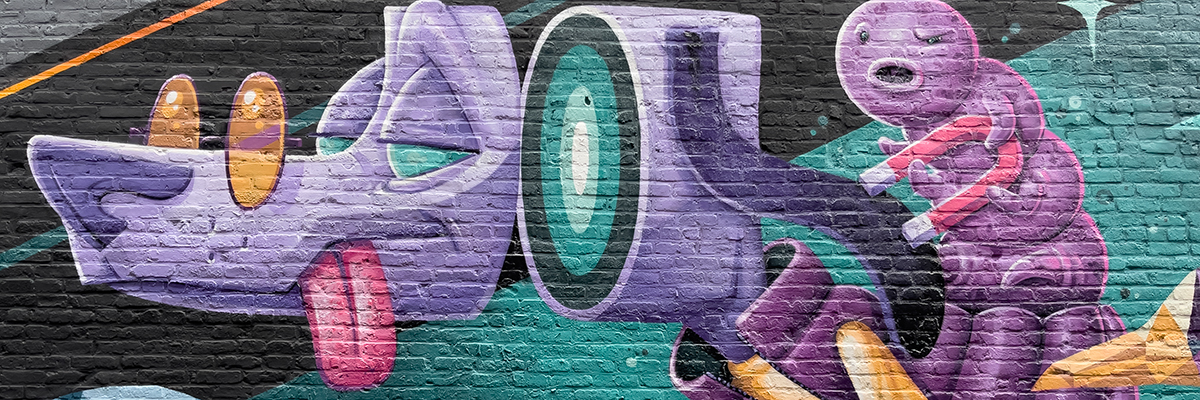This vibrant and highly stylized mural, painted on a brick wall, spans a wide, thin rectangle. The background features a diagonal composition consisting of a teal stripe running from the upper right to almost the lower left, overlaid with a black stripe. Dominating the left side of the image is a robotic dog head, which is purple with teal eyes and wears distinctive yellow-tinted, circular glasses reminiscent of Ozzy Osbourne's iconic eyewear. The dog's mouth is agape, revealing an extended pink tongue. Notably, the back of the dog's head is artistically depicted as cut and floating, exposing a circular cross-section of its mechanical interior. Attached to the dog's head is a peculiar purple, worm-like figure with multiple arms, a round head, and an oval mouth, holding a U-shaped magnet as it appears to interact with the dog's ear. This captivating blend of whimsy and surrealism, executed with meticulous detail, creates an engaging visual narrative on the urban canvas.